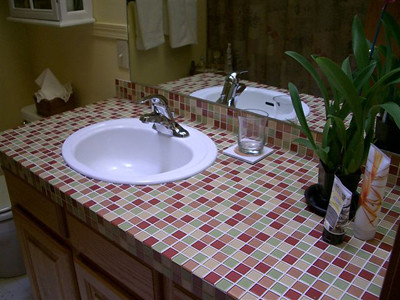This image depicts a quaint bathroom setting. The countertop is adorned with a mosaic of tiles in varying hues—green, red, light red, and pink—randomly arranged to create a colorful, eye-catching surface. A pristine white sink, complete with a sleek metal faucet, is positioned centrally on the counter, its reflection clearly visible in the mirror above. In the mirror, portions of the colorful tiles and additional mirrors placed behind the sink also come into view.

To the right of the sink, a lush green plant adds a touch of nature, while several containers holding various items are neatly arranged nearby. On the left side of the image, near the upper part of the wall, a white cabinet offers storage. The wall itself is painted a soft cream-yellow, providing a warm backdrop to the room's features.

In addition, a brown basket filled with white items sits adjacent to the tiled counter, contributing to the room's cozy feel. The lower portion of the image reveals a glimpse of the floor and a glass placed on the countertop. Beneath the glass, a white square, possibly a coaster, is apparent, along with its faint reflection. This bathroom blends functionality and aesthetic appeal, featuring a rich array of textures and colors.